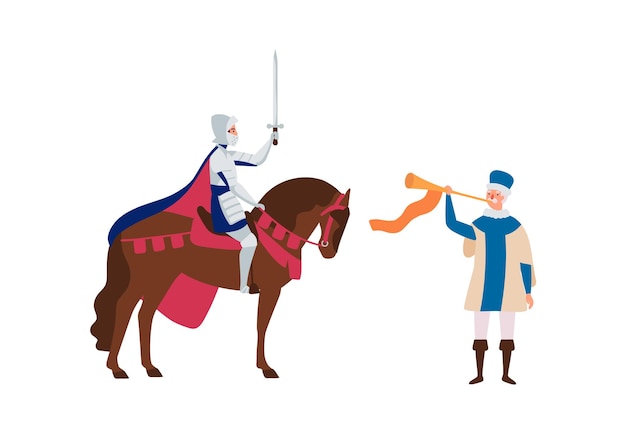The image depicts a detailed clip art-style illustration with a white background. On the left side, there's a tall, medium-brown horse facing to the right. The horse has darker brown mane and tail, and is adorned with red gear and pink banners. Mounted on the horse is a knight in full silver armor, including a helmet, and a blue cape with red and pink lining. The knight is holding a white sword with a brown handle upright in his left hand. 

On the right side of the image is an older white man with white hair, wearing a cream and blue tunic, white pants, and brown knee-high boots. He is blowing an orange trumpet with an orange flag attached. A blue cap adorns his head. The scene captures a moment of interaction between the knight and the bugler, with the trumpet being played in the direction of the knight.